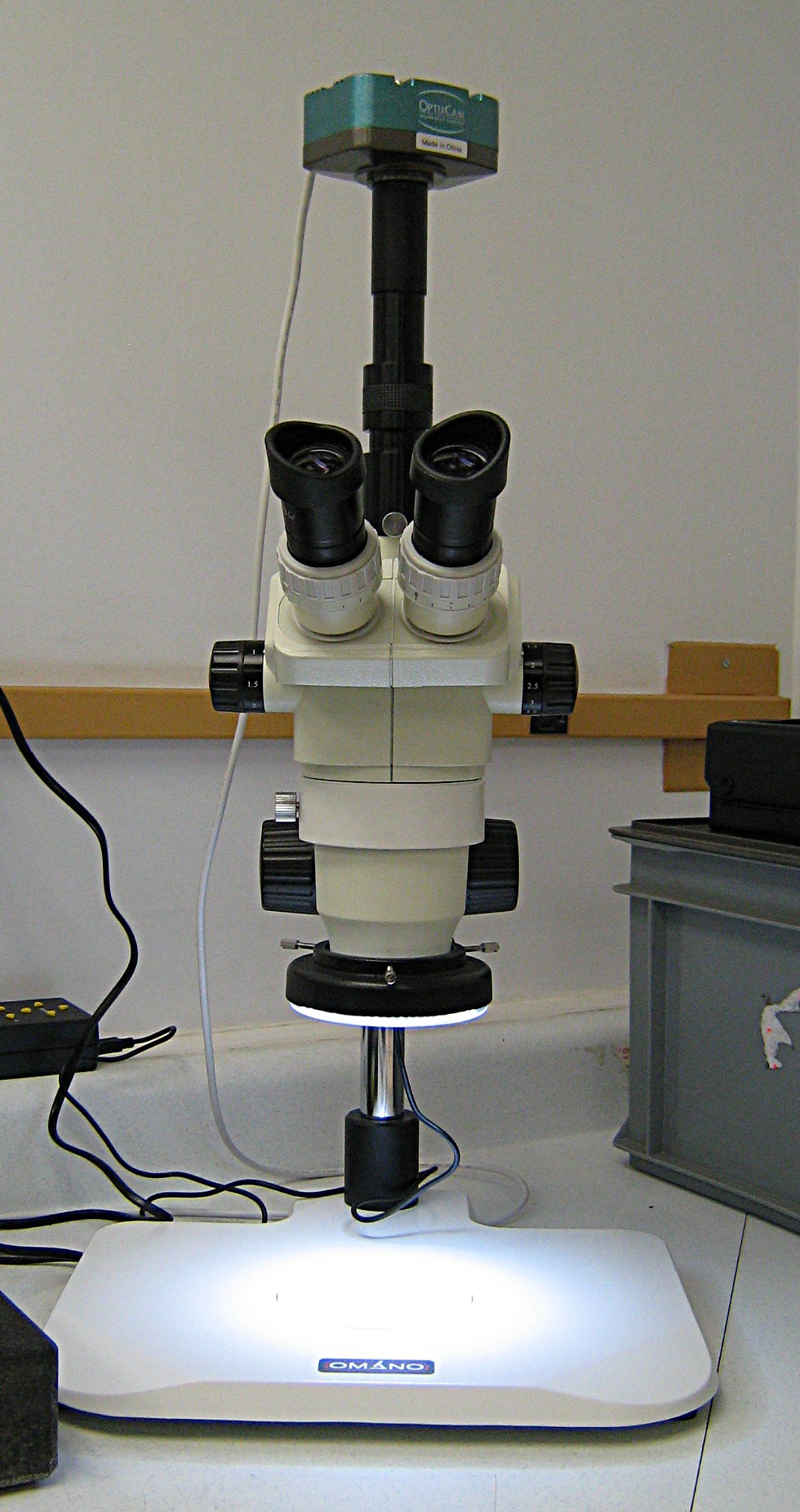The indoor image depicts a detailed setup used in a hospital or optometrist's office, featuring specialized equipment on a white countertop with black trim. At the center, there is a sophisticated microscope with a large viewing area on top that includes green accents. The setup includes a prominent base and appears intricate, probably used for examinations such as checking for germs or analyzing the details of an eye test. The background consists of white walls with a section of wood trim, and the workspace includes various scattered equipment and cords. Notably, to the left of the microscope, there is a power strip with a cord, and to the right, a gray box with a black box placed on top of it.